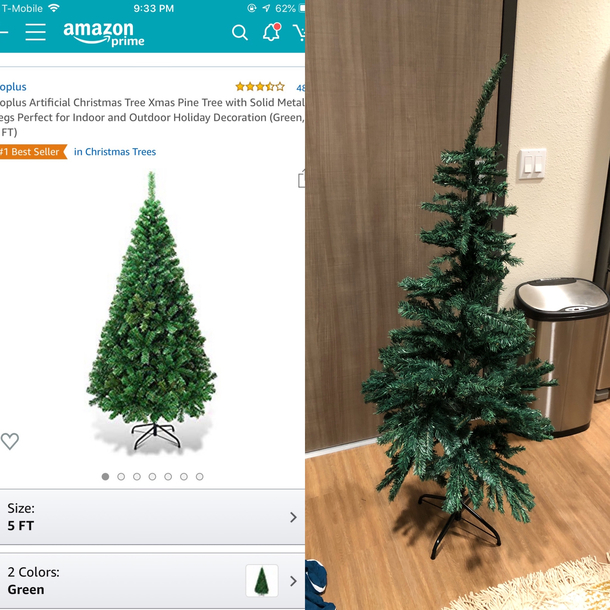Here's the cleaned-up and detailed caption for the image:

---

This image features two side-by-side screenshots from a phone showcasing an Amazon Prime Shopping interface. 

**Left Screenshot:**
- **Header:**
  - A blue border with white lettering at the top, displaying "T-Mobile" on the left.
  - Wi-Fi icon, current time at the center, and battery percentage with an upward arrow on the right.
- **Main Interface:**
  - Under "T-Mobile," three white lines are visible, indicating a menu.
  - Amazon Prime logo with a white checkmark is prominently displayed.
  - Icons for search and notifications are located beside the logo.
  - A partial view of an item card browsing Christmas trees, with the left side cut off.
  - Visible partial text in blue showing "O-P-L-U-S," and a rating of three and a half stars.
  - An orange label indicating "No. 1 Best Seller" in white text is to the right.
  - Blue text reads "in Christmas trees."
  - Below this is an artificial Christmas tree description.
  - Interface elements include a gray circle followed by five white circles with gray borders.
  - Two gray tabs below: the left one indicating "Size" with "5 feet" and the right one showing "Two colors" with "Green."

**Right Screenshot:**
- A stark contrast with a depressing-looking Christmas tree that appears unkempt and sparse.
- The tree has significantly fewer branches than the one on the left side.
- The tree is standing on a wooden floor in front of a wooden door.
- To the right of the tree, a portion of a white wall and a silver trash can at the base are visible.

---